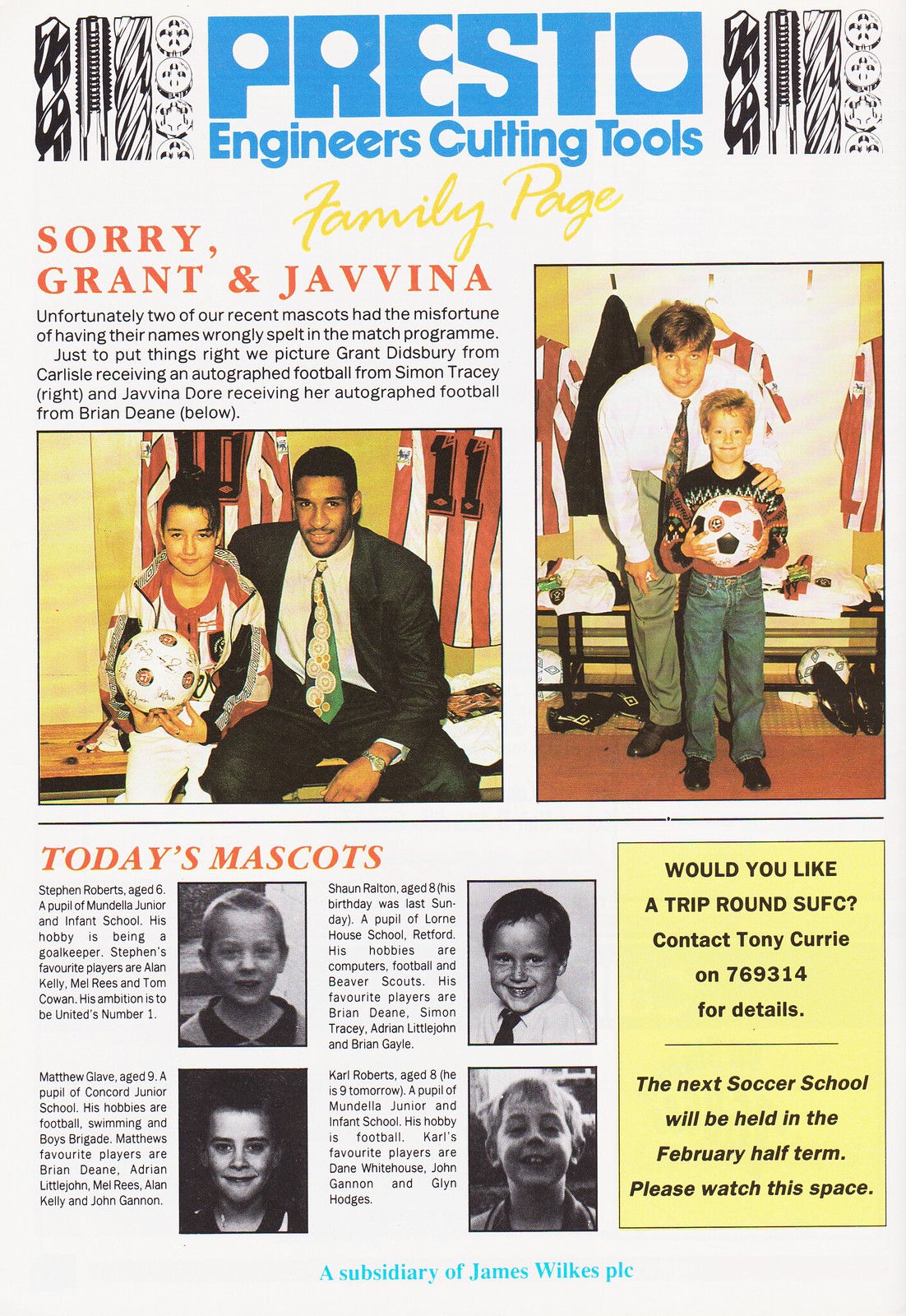This page from a magazine illustrates a detailed and heartfelt family-centered segment by Presto Engineers Cutting Tools. The top of the page prominently displays the brand name, "Presto Engineers Cutting Tools," with intricate tool drawings interspersed among the words. Just below this, in yellow cursive text, is the label "family page," suggesting a corporate magazine feature focusing on employees and their families.

In a striking red font, it reads "Sorry, Grant and Jovina," followed by an explanation in black text: "Unfortunately, two of our recent mascots had the misfortune of having their names wrongly spelled in the match program. Just to set things right, we picture Grant Didsby from Carlisle receiving an autographed football from Simon Tracy Wright, and Jovina Doerr receiving her autographed football from Brian Dean Below."

Accompanying this text are photos: on the left, a girl named Jovina happily receiving an autographed soccer ball from Brian Dean, and on the right, a boy named Grant being similarly honored by Simon Tracy Wright. These images highlight the joy and rectification of the error.

The lower part of the page, titled "Today's Mascots," features black-and-white close-up photos of other children mascots, complete with informative captions about each. On the far right, a yellow box advertises a special offer: "Would You Like a Trip Around SUFC? Contact Tony Kareen," suggesting an interactive element for the readers.

The page's theme is predominantly soccer-related, with a variety of colors such as yellow, white, blue, black, red, brown, cream, and tan enhancing the visual appeal. The photos and the layout suggest an indoor setting, reinforcing the magazine’s polished, professional vibe. All in all, this magazine page provides a rich tapestry of corporate pride, family values, and community engagement.